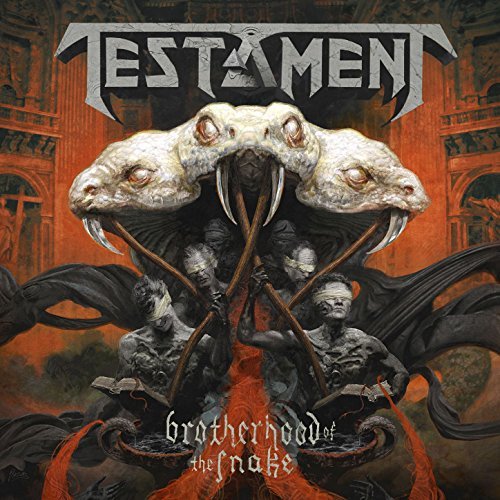The image appears to be an ornate and dramatic cover, likely for an album or CD by the band Testament. It features a prominent background of an orangish-brown hue, resembling the interior of a grand cathedral or a music auditorium with gray, dark, smoky, and red Romanesque columns. Dominating the middle of the image are bold, gray letters spelling "Testament." Below this title, a white three-headed snake with long fangs is depicted. Emerging from or being devoured by the snake’s mouths are six blindfolded, gray-skinned, devilish-looking figures. These figures are holding large, thick books and sticks, seemingly keeping the snakes' jaws open. Surrounding these figures is a flowing, membrane-like or fibrous structure, adding to the chaotic scene. At the very bottom of the image, the text "Brotherhood of the Snake" is displayed in ornate white lettering against a smoky backdrop, enhancing the dystopian and haunting atmosphere of the artwork.